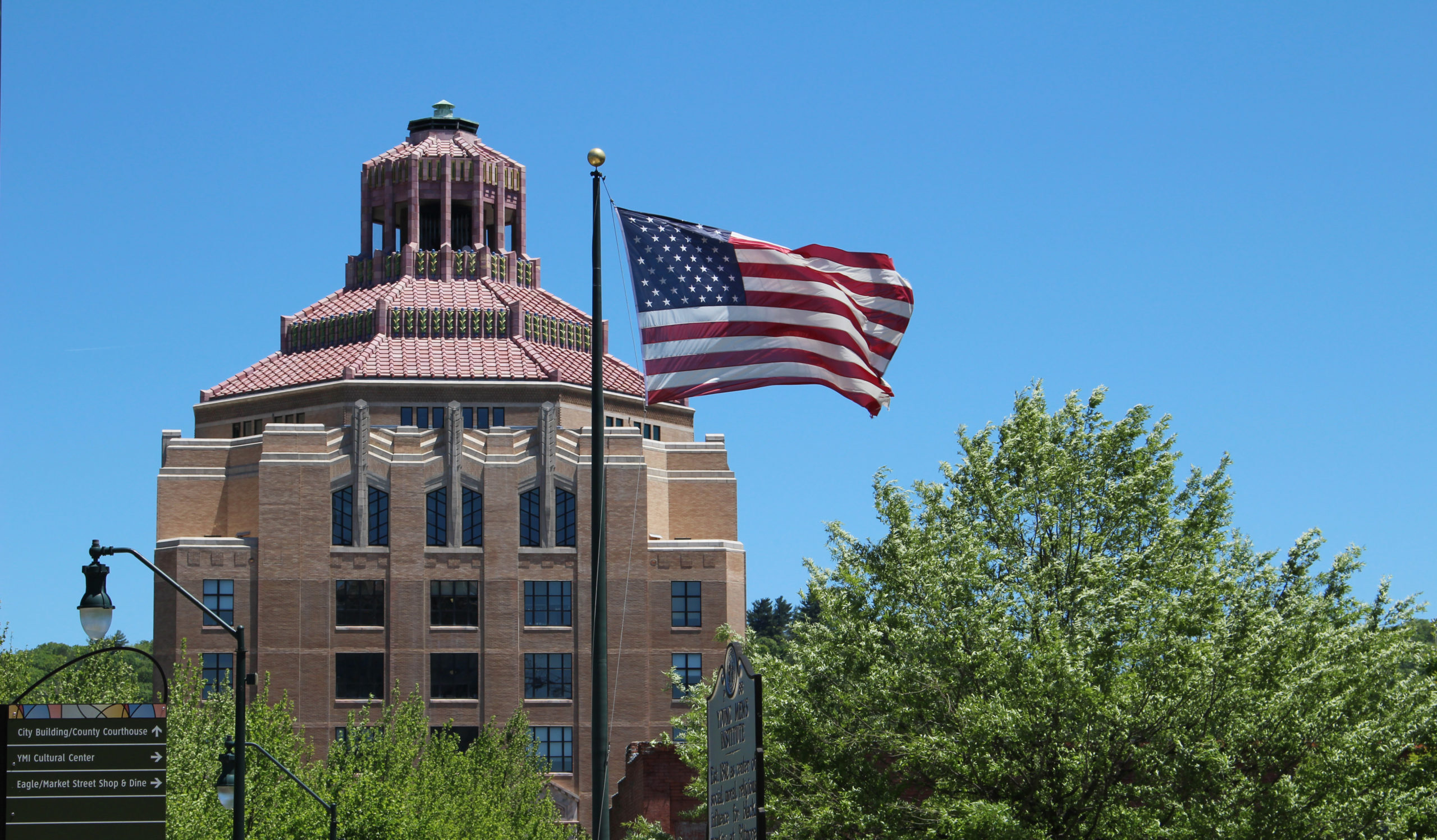The photograph captures a bright, sunny day with a clear, vibrant blue sky devoid of clouds. Dominating the scene is a multi-level, sandy-colored brick building with numerous windows and a distinctive multi-tiered, almost conical red roof. Adorning the facade is a lookout at the top, which is currently unoccupied. In the foreground, several leafy green trees partially obscure view of the building, while prominently displayed is an American flag waving proudly on a flagpole. The flag showcases its characteristic red and white horizontal stripes and a blue square studded with white stars. To the left, an assortment of street lights and directional signs are visible. One sign, bearing black and white text, directs to the "City Building / County Courthouse" with an arrow pointing upwards, and to the "Cultural Centre" and "Eagle / Market Street Shop and Dine" with arrows pointing to the right. The skyline in the distance is a continuous row of trees, creating a serene backdrop for the bustling area in the foreground.